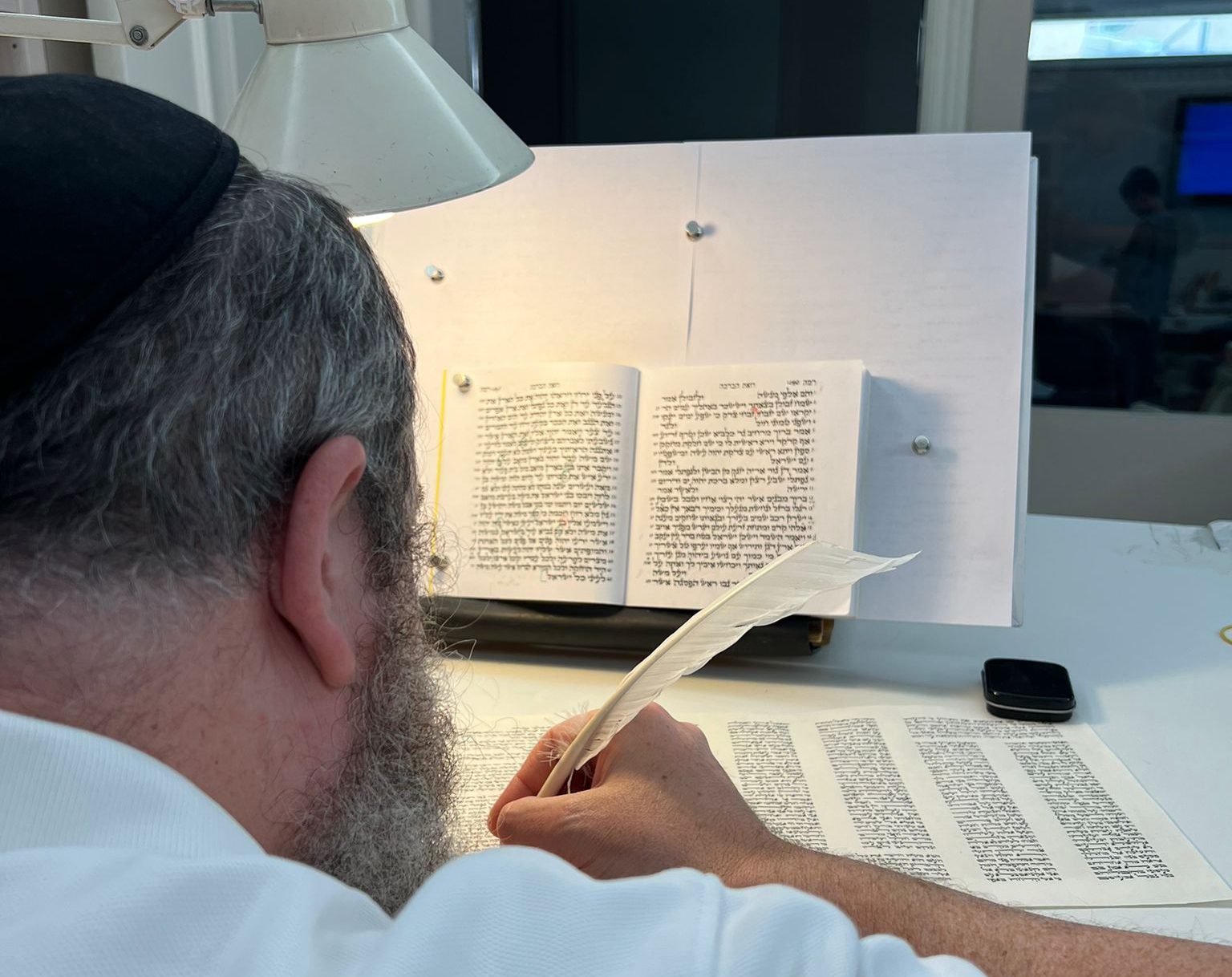The square, full-color indoor photograph, illuminated by artificial light, captures a detailed and serene scene focused on a Jewish man engaged in writing. The man appears aged, evidenced by his grey hair and beard accented with white streaks. Clad in a white shirt and wearing a yarmulke slightly tilted to the left, he is visible from behind, showcasing his right shoulder, ear, and side profile. His right arm is extended as he uses a white quill pen to write meticulously on a sheet of paper. The text he is writing is in fine, likely non-English print, suggesting Hebrew. In front of him, a book is positioned upright on a book holder, propped to remain open. This book, also illuminated by a lamp above it, seems to be the source he is transcribing from, with its text appearing in black ink. The desk below is white, and a slim black box with a white outline sits to the bottom right of the book holder, adding a subtle detail to the composition. The overall scene suggests a moment immersed in scholarly or religious study.